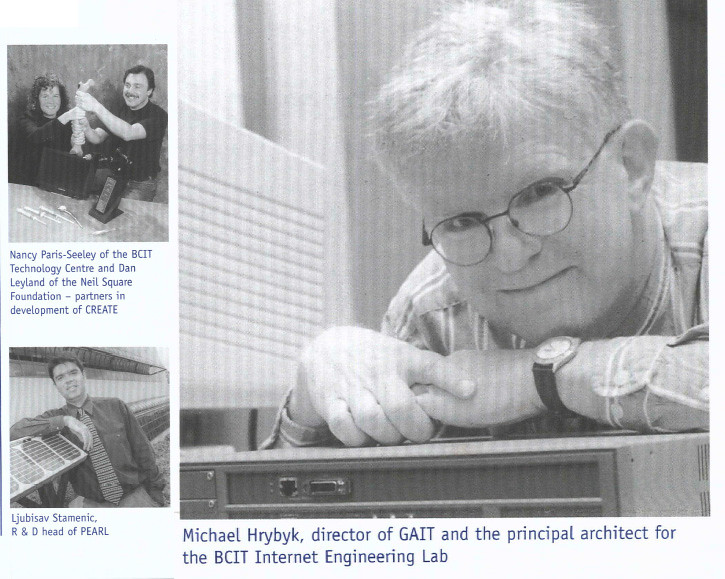The image is a meticulously designed black-and-white photographic representation, evoking a sense of realism and precision. It comprises three distinct photographs arranged in a landscape orientation, portraying key individuals involved in an engineering project. Dominating the right two-thirds of the composition is a large, square-format portrait of an elderly man with white hair and wire-rimmed glasses, named Michael Hribek. He is seen smiling and looking up at the viewer, with his hands folded over an electronic piece of equipment. He is dressed in a light-colored striped dress shirt and wears a watch on his left wrist. The caption below his photograph reads: "Michael Hribek, director of GATE and the principal architect for the BCIT Internet Engineering Lab."

On the left side of the layout, there are two smaller, vertically-stacked photographs. The upper photograph features a young woman with curly hair and a younger man with a mustache, both smiling and holding an object up. The caption beneath it identifies them as Nancy Parasili of the BCIT Technology Center and Dan Leyland of the Neal Square Foundation, partners in the development of CREATE. The lower photograph depicts a man in a business shirt and tie, leaning on a piece of equipment and smiling, identified as Lujubzev Stamenik, R&D head of Pearl. The cohesive combination of photographs and carefully arranged typography on the page detail highlights the collaborative efforts of these individuals in their respective technological and engineering fields.